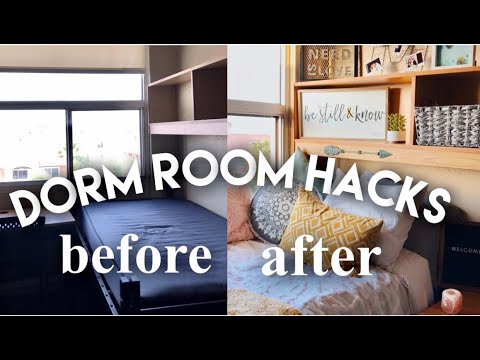This image, likely a YouTube thumbnail titled "Dorm Room Hacks," features a striking side-by-side, split-screen comparison of a dorm room before and after decoration. On the left side, the "Before" picture displays a barren dormitory with only a blue twin-size mattress, devoid of any personal touches, including the empty desk and bookshelves. The right side, labeled "After," showcases the transformative power of decor, with the same space now fully furnished and vibrant. The bed is adorned with several pillows and blankets, while the previously empty shelves are now filled with various decorations and personal items. Text overlaying the image clearly marks the transformation, highlighting the impact of dorm room hacks in creating a warm, personalized living space.